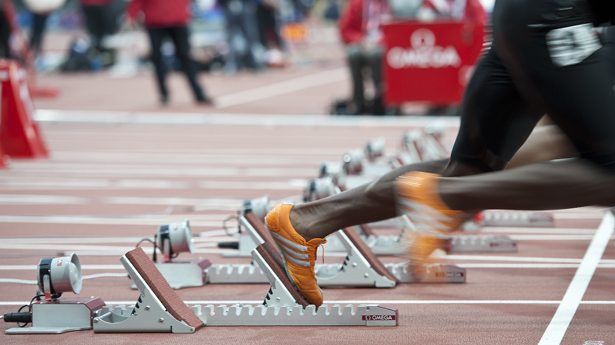The photograph captures the electrifying start of a sprint race, likely at a professional or Olympic-style event. The image vividly shows the runners at the starting line, having just launched off their springboards, also known as starting blocks, which are crucial for ensuring a fair and powerful takeoff. Foremost in the frame is an athlete sprinting forth with notable intensity. He is distinguished by his neon orange Adidas sneakers, adorned with white stripes, and he appears to be of African descent. His athletic attire includes tight, black running shorts with a white patch on the side. The motion blur in his legs underscores the action and speed of the moment, emphasizing that he has just taken off. The backdrop features blurred figures of other runners, coaches, and possibly referees or judges, all contributing to the race's official ambiance. Additionally, there's a red table with individuals in red shirts, symbolizing race officials, and a red square with a white emblem, likely representing the event's branding. The setting is a running track with spectators and officials intently observing the race commencement.